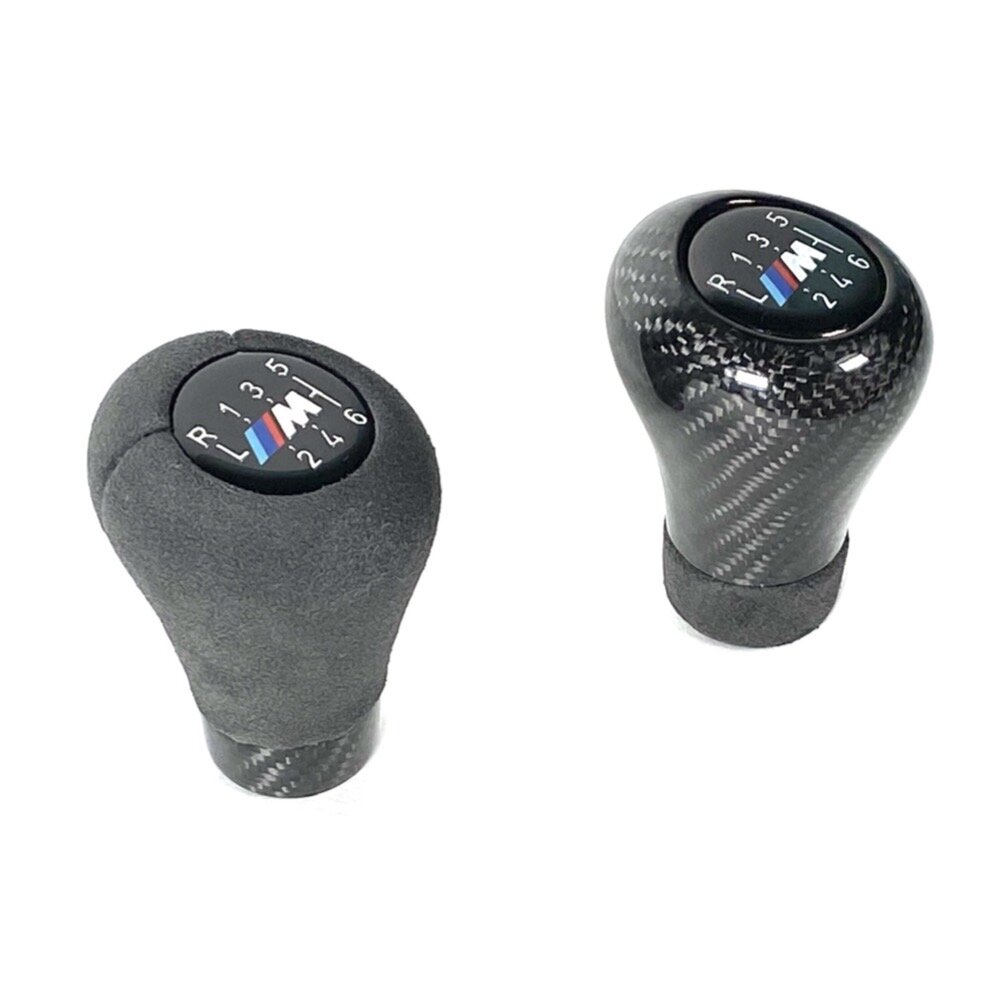The image displays two car shifter knobs against a pristine white background. The knob on the left features a soft, gray fabric material enveloping its majority, with a distinct strip of carbon fiber-like material at the bottom. At the top center, the knob boasts a plastic-covered dial indicating the gear positions: R, 1, 3, 5 at the top, and 2, 4, 6 at the bottom, prominently displaying an "M" logo comprising light blue, dark blue, red, and white colors, arranged in a rhombus shape. The counterpart on the right is essentially the reverse in design, predominantly showcasing a sleek, carbon fiber-like finish, complemented by a strip of the same gray fabric material at the bottom. This knob also features the same plastic dial at the top, detailing the gear positions R, 1, 3, 5, and 2, 4, 6 beneath, with the identical multicolored "M" logo in the center.